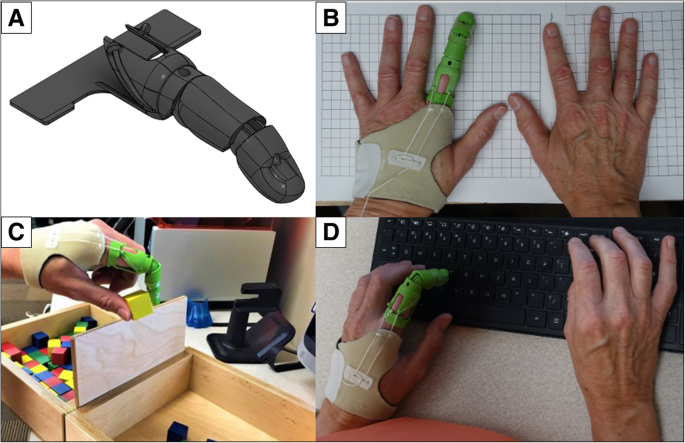The image is a four-part photo grid demonstrating the use of an index finger prosthetic. The top left image (A) is a digital representation of the prosthetic, showcasing a black or dark-colored artificial finger. Adjacent to it, the top right image (B) features a photograph of two hands stretched out on graph paper, with the left hand fitted with a green prosthetic finger. The bottom left image (C) captures a hand with the prosthetic transferring a toy block from one box to another. Finally, the bottom right image (D) depicts two hands typing on a keyboard, with the left hand wearing the prosthetic, effectively illustrating its functionality in daily activities.